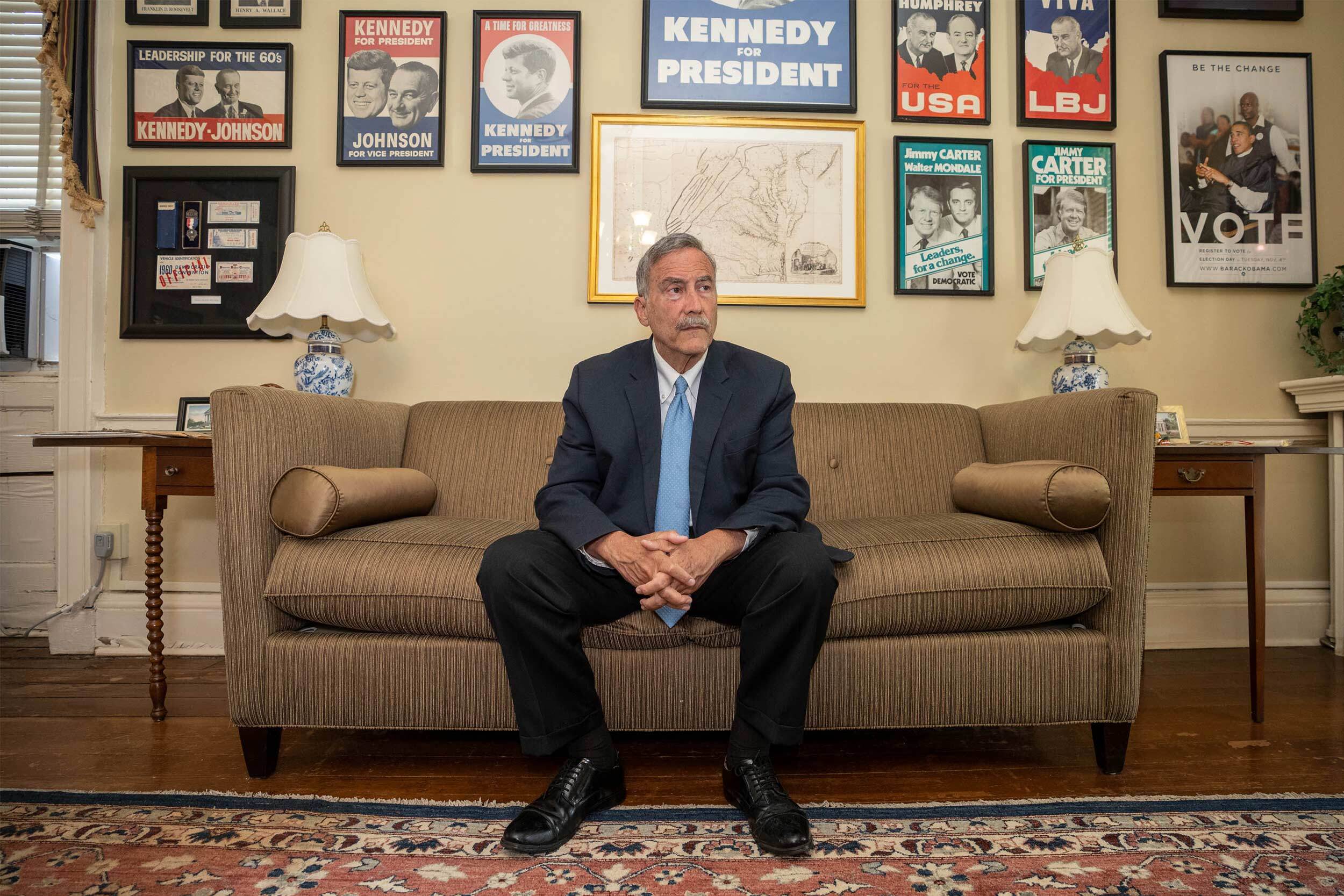In this detailed image, a man with short gray hair and a silver mustache sits on a light brown couch that features thin vertical stripes and appears to be made of a smooth satiny material. The couch, large enough to seat two or three people, has two small round pillows, one on each side. Clad in a blue suit jacket, a white shirt, a light blue tie, black pants, and black dress shoes, the man leans forward slightly, resting his elbows on his thighs and gazing off to the side with a serious expression.

The couch is flanked by small wooden end tables, each holding a lamp with a blue and white base and a cream-colored shade. The floor beneath the man's feet is covered by a red, beige, and blue carpet, which lies on a visible brown wood floor extending from the left to the right under the couch.

Behind him, a beige wall is densely decorated with a collection of framed political posters, primarily featuring slogans like "Kennedy for President." Several posters promote John F. Kennedy with variations such as "A Time for Greatness" and "Kennedy for President, Johnson for Vice President." Other posters on the wall endorse Jimmy Carter and Walter Mondale, with slogans such as "Leaders for a Change" and "Vote Democratic." The room exudes a strong historical and political ambiance.